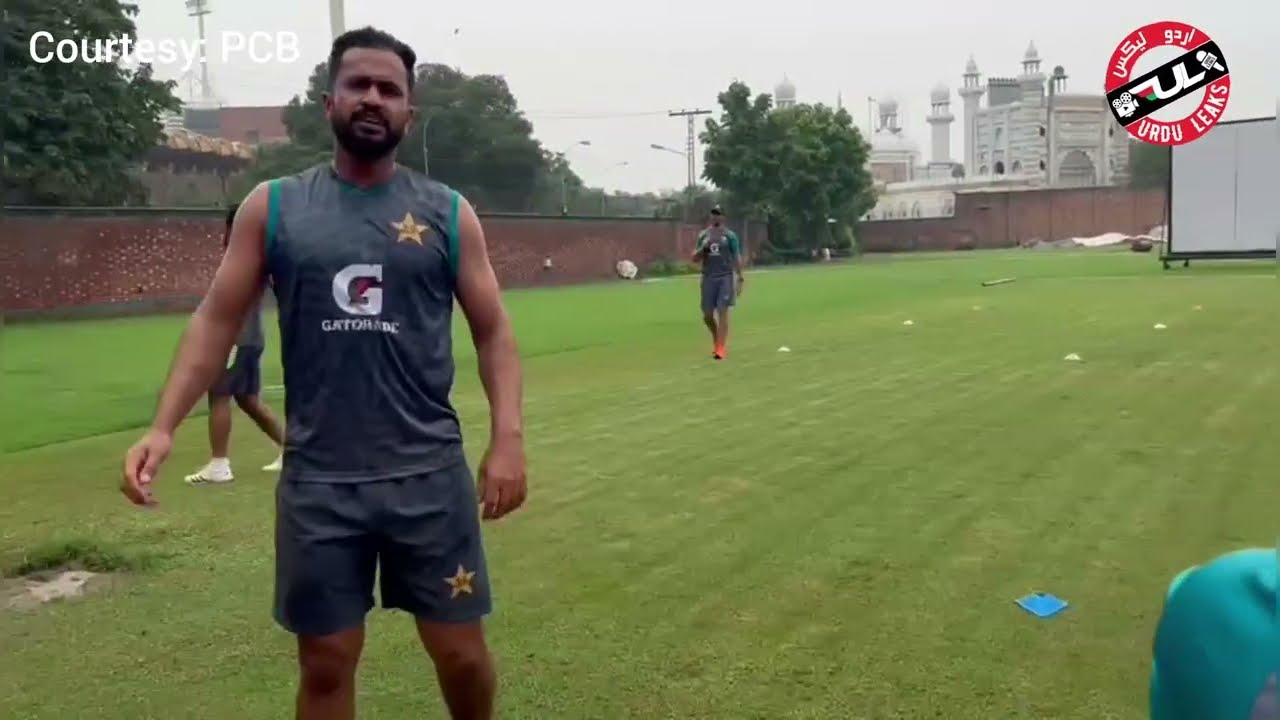In an overcast outdoor setting, a photograph captures a muscular, dark-skinned man standing on a grassy soccer practice field, wearing a gray, sleeveless uniform adorned with the Gatorade logo and stars on both his shirt and shorts. His attention seems directed towards the camera. To his left, another man in a similar uniform with orange shoes walks into the frame from the left side, while a third person, partially obscured, heads rightward. The field is marked with small practice cones and bordered by a large red brick wall. In the background, a white mosque with several tall towers is visible, adding a striking architectural element to the scene. The sky is cloudy, and trees partially surround the wall. At the top of the horizontal rectangular image, white text reads "Courtesy: PCB," while the upper right corner features a red circular logo with "URDU leaks" inscribed.